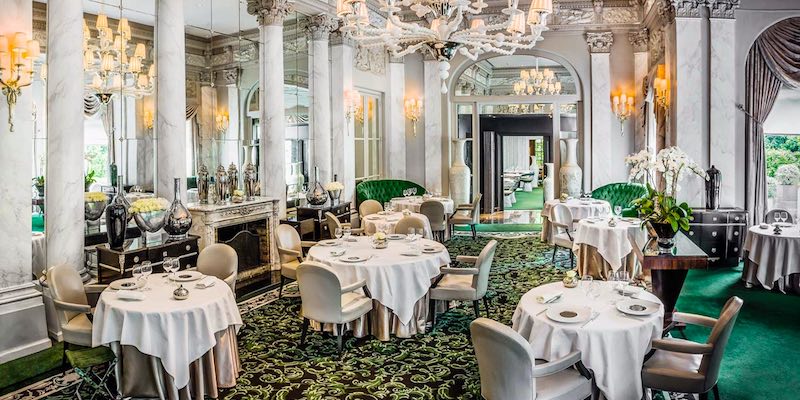The illustration depicts an exquisitely detailed and ornate dining room that exudes elegance and luxury. There are approximately nine round dining tables, each draped with pristine white tablecloths and meticulously set with fine silverware, plates, and wine glasses. Most of the tables are surrounded by cushioned chairs with armrests, while a few also feature cozy couches. The room is adorned with marble columns and mirrored walls, enhancing the grandeur of the space. 

On the left side, a stately fireplace adds a quaint touch, while a large chandelier descends from the ceiling, casting a soft glow over the scene. The floor is covered with an intricate art deco carpet featuring dark brown, black, and green patterns of crawling vines and leaves. A green lounge chair rests on the right-hand side, next to large vases flanking a black doorway that leads to another room. The backdrop of the room includes several elaborate chandeliers and decorative elements, contributing to the overall opulence. This beautifully illustrated dining hall could easily belong to a high-end restaurant or a grand mansion, showcasing an unforgettable, luxurious ambiance.